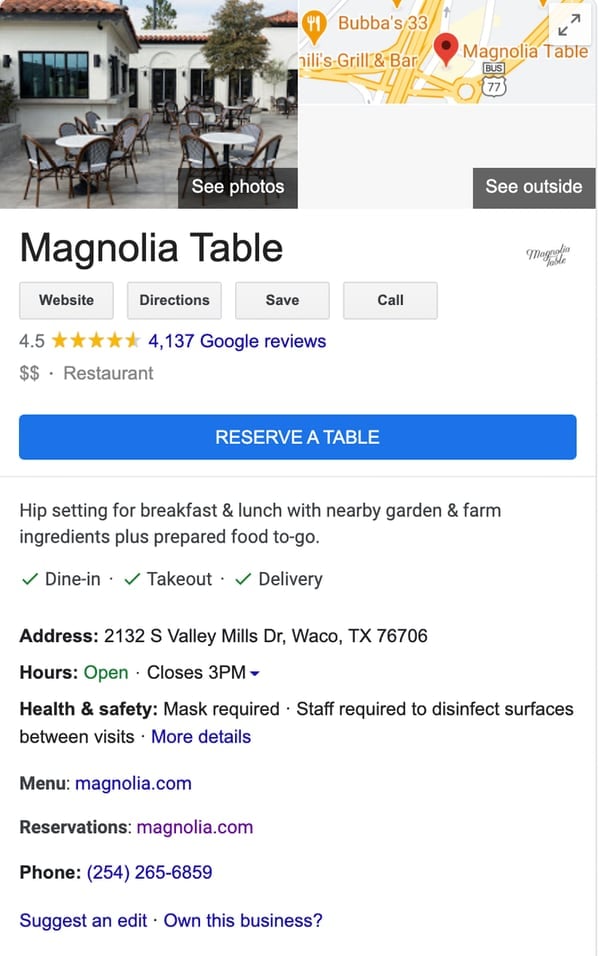This detailed caption provides an elaborate overview of an online listing for a restaurant named Magnolia Table:

---

**Magnolia Table Restaurant Overview**

At the top of the listing, a vibrant image of an outdoor patio at Magnolia Table sets the scene, exuding a cozy and inviting biophilic atmosphere perfect for dining. A semi-sheer black rectangle overlay suggests viewing additional photos of the establishment.

Adjacent to the image is an interactive map, with a gray rectangle offering a sneak peek of the exterior through the "See Outside" option.

Directly below the image, the restaurant's name, *Magnolia Table*, is prominently displayed. Four functional gray buttons beneath this include options to visit the restaurant's website, get directions, save the listing, and make a call to the establishment.

The restaurant boasts a stellar rating of 4.5 out of 5 stars, based on an impressive 4,137 Google Reviews, represented by five bright yellow stars and blue digits. Priced moderately, as indicated by two dollar signs, Magnolia Table caters specifically to breakfast and lunch crowds with an emphasis on using nearby garden and farm ingredients. Additionally, they offer prepared food to go.

A blue "Reserve a Table" button stands out, inviting customers to secure a spot at the restaurant. Below, a light gray line separates this from further details about the dining experience.

A concise description outlines the restaurant's atmosphere as a "hip setting for breakfast and lunch" where local ingredients are featured, including options for [**dine-in** green checkmark], [**take-out** green checkmark], and [**delivery** green checkmark].

Further down, precise address details and operational hours are provided, indicating the restaurant is indeed "open" with a note that it closes at 3 p.m. Health and safety measures include a requirement for masks and a mandate for staff to disinfect surfaces between visits. More extensive details are accessible via a blue "More Details" link.

Additional options like the menu are also available, with links to their website and reservation page, along with contact information displayed in blue and purple fonts.

Concluding the listing are options to suggest an edit or claim ownership of the business under the prompt "Own this business?"

---

This comprehensive description helps potential diners get a clear, thorough understanding of what Magnolia Table offers and how to interact with their services and information.